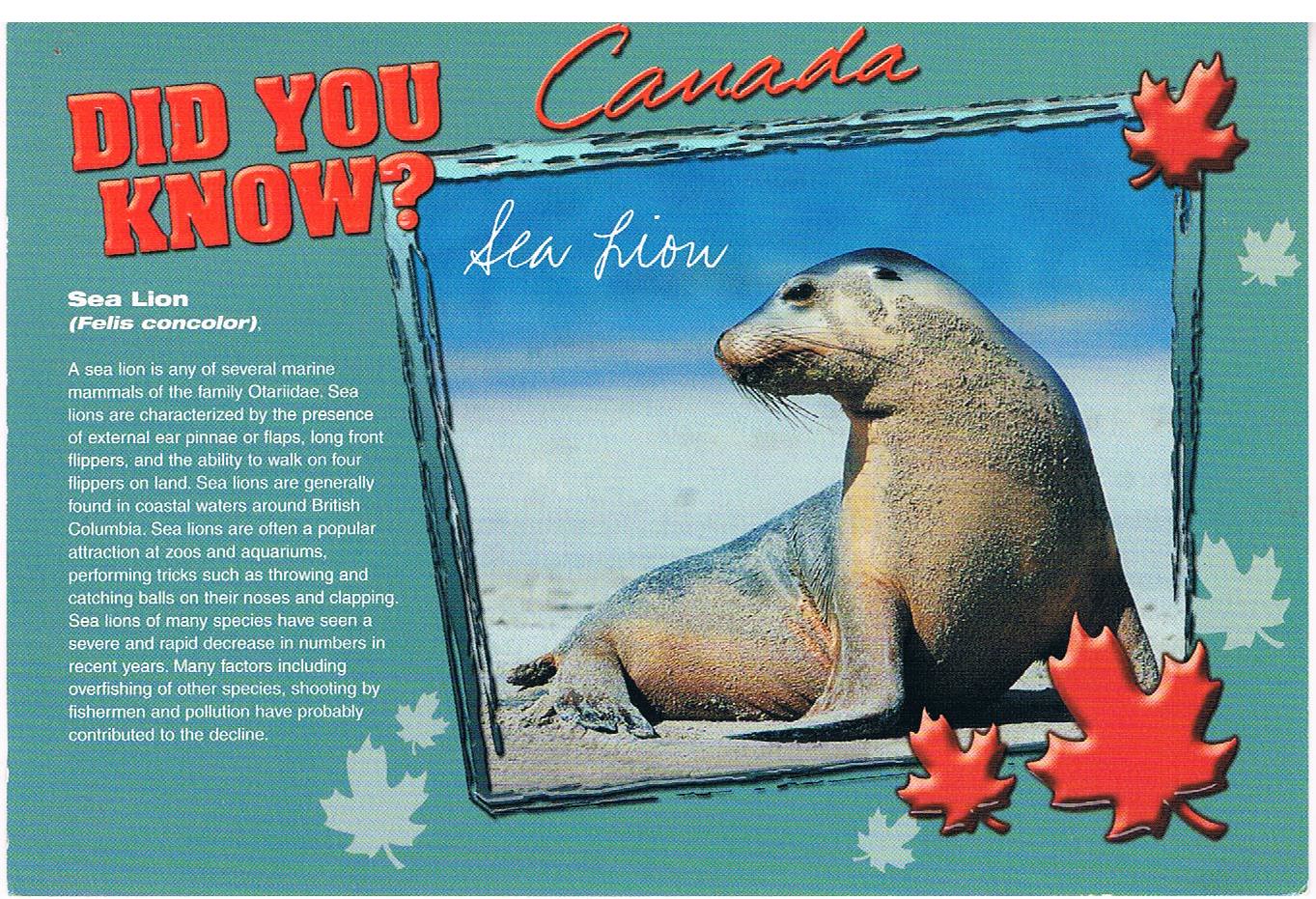The informational flyer prominently features a photograph of a sea lion lying on sandy beach, gazing to its left, with sand covering parts of its body. Encased within a blue border adorned with three red maple leaves on the top right and two on the bottom left, the image is labeled "Sea Lion" in elegant white cursive font in the top left corner. Adjacent to the photograph, a body of white text on a blue background details the animal: "Sea Lion Felis Concolor. A sea lion is any of several marine mammals of the family Otariidae. Sea lions are characterized by the presence of external ear pinnae or flaps, long front flippers, and the ability to walk on four flippers on land. Sea lions are generally found in coastal waters around British Columbia." Above the text, bold red letters spell out "Did you know," adding an informative touch to the flyer, which is styled to showcase Canadian pride with its consistent maple leaf design.